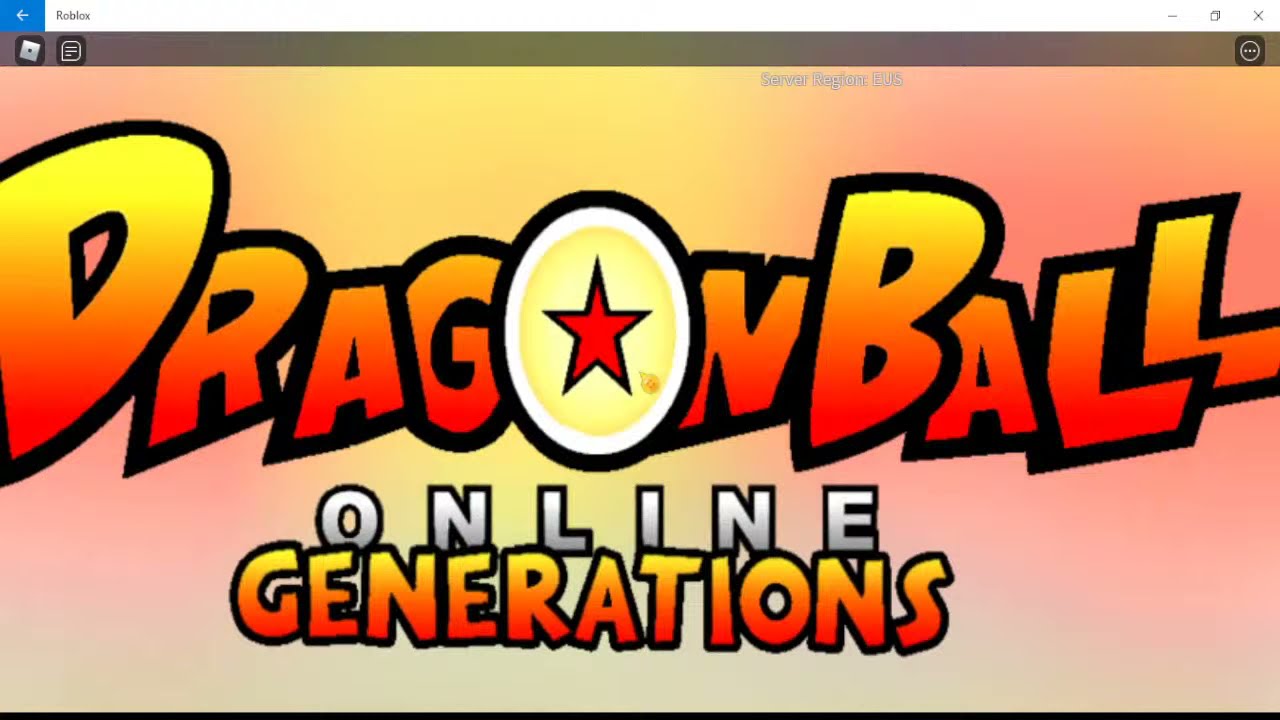The image is a graphical logo set against a multicolored gradient background featuring alternating shades of yellow and red, resembling a sunset. In the center, the words "Dragon Ball" appear in large, bubbly, all-caps text with a bold gradient effect transitioning from yellow at the top to red at the bottom, outlined in black. Notably, the 'O' in "Dragon" is replaced by a yellow circle containing a red star, reminiscent of an emblem. Below "Dragon Ball," the word "Online" is written in light gray, capital letters with a black outline. Further down, the word "Generations" follows the same gradient color scheme as "Dragon Ball," starting with yellow at the top and fading into red at the bottom, also outlined in black. The background also includes a blue back button and the word "Roblox" in the upper left-hand corner within a white header bar, along with typical computer interface elements like an X and screen resize button in the top right. At the bottom of the image, there's a small gray rectangle and an adjacent white rectangle containing part of a computer user interface.